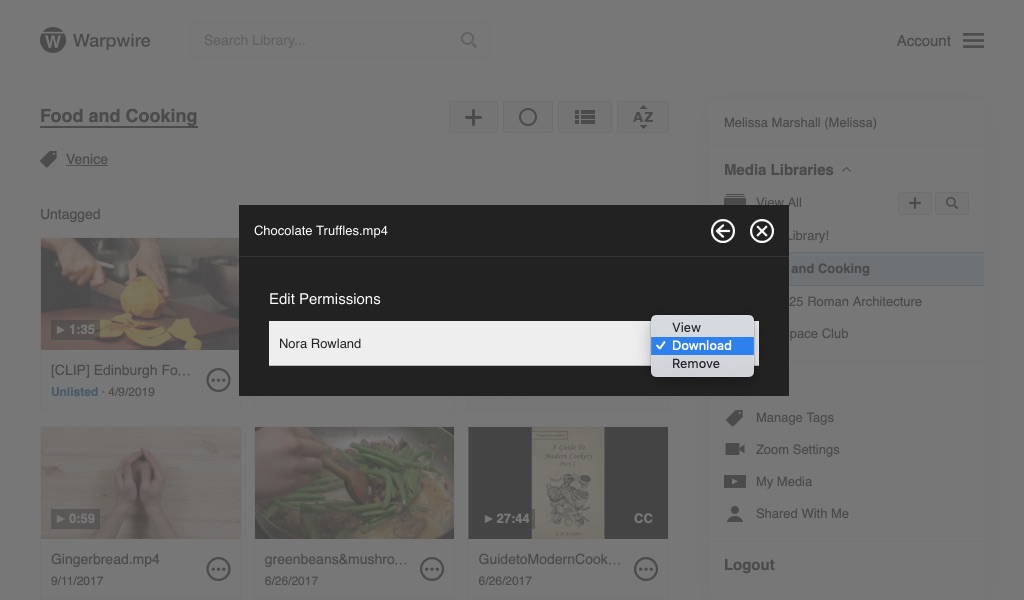The image showcases a screenshot of a webpage from Warpwire, identified by a black circle with a white "W" in the upper right-hand corner. The interface features a search library section on the left, and a user account detail area on the right. Directly beneath this are labels for categories including "Food and Cooking," "Venice," "Untagged," and more. Several video thumbnails are visible at the bottom, displaying tutorials such as "How to Make Gingerbread" and "How to Make Green Beans and Mushrooms," among others.

The background of the screen appears slightly muted or grayed-out, indicating an overlay. This overlay presents a black rectangle at its center, prominently displaying the file "chocolate truffles.mp4." Below the file name, options for "Edit Permission" and the name "Nora Rowland" are visible. Additional interactive elements include buttons labeled "View," "Download," and "Remove." In the top area of the overlay are navigation options, featuring both a back button and an "X" icon to close the popup. The visible activity suggests the user is currently in the process of downloading the file, "chocolate truffles.mp4."